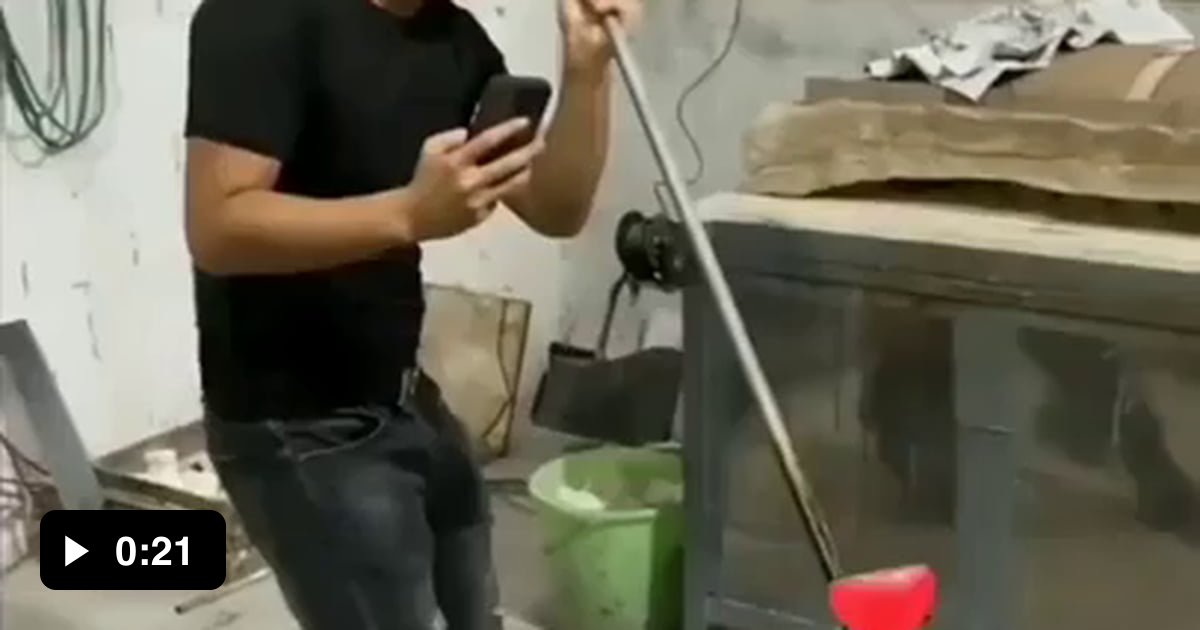In the image, there is a white Caucasian individual standing with a black t-shirt and dark grey jeans. The person is holding a green pole and a black phone in their left hand. To the bottom left of the image is a black square with a white triangle pointing to the right, indicating that this is a video of 21 seconds duration. At the base of the green pole, there is a red object. Behind the person, the off-white walls feature a red cord along the perimeter and a black cord hanging behind them. Near the individual's leg, there is a small green bucket. The flooring in the scene is grey, and the siding along the bottom part of the wall appears to be a darker grey. Additionally, there is a brown item leaning against the wall.